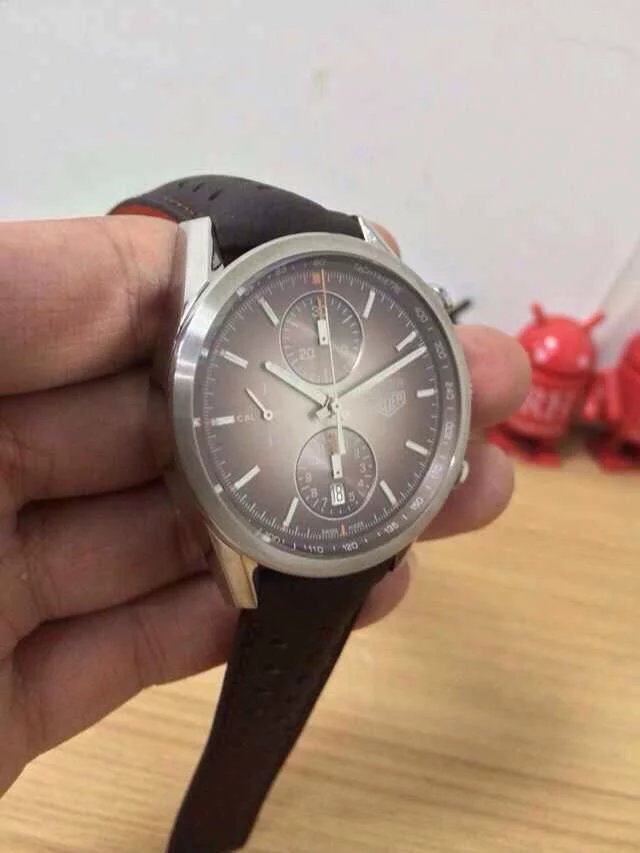In this photograph, the backdrop features a white upper wall transitioning into a rich golden brown hardwood floor. The right side of the image showcases two small, red-painted plastic robots with antennas protruding from their heads, resembling alien figures. On the left, a person's light-complexioned hand extends into the frame, palm unseen, with four fingers visible. Draped over these fingers is a black leather-strapped watch. The watch's face is round and silver, displaying the time as 11 minutes past 10, and the date as the 18th. Its minimalist design features lines representing the hours, with two additional sub-dials above and below the hands, potentially indicating various functions. The scene is set on a surface that could be interpreted as a desk or table, complementing the robots and emphasizing the primary subject—the intricately detailed watch and hand.